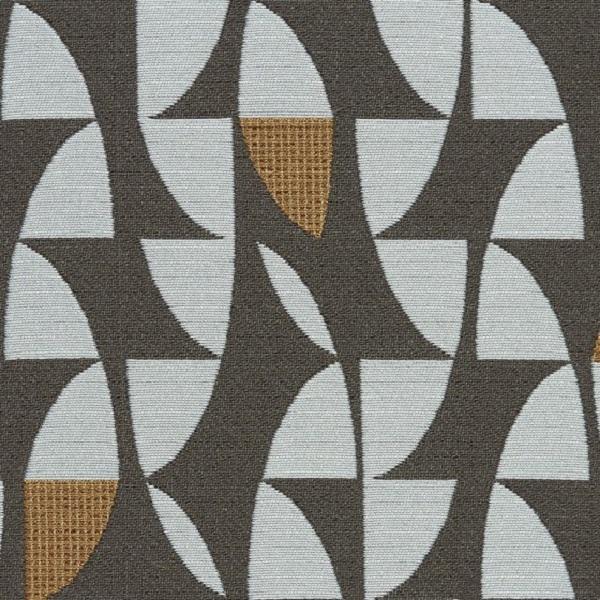This commercial photograph showcases a square-shaped rug, designed with a striking abstract pattern ideal for online retail or catalog listings. The rug's surface features interchanging dark gray, light gray, and brown motifs arranged in a somewhat random sequence. These alternating patterns give it a dynamic, textured appearance. Additionally, there are noticeable tan patches woven into the fabric, reminiscent of burlap, adding a touch of rustic charm. The intricate design includes abstract shapes that resemble leaves or plant life, creating an organic feel amidst the geometric layout. The fabric itself appears coarse, highlighting the quality and durability of the material used in the rug. This rug's blend of gray shades and abstract patterns makes it a versatile accessory for various interior styles.